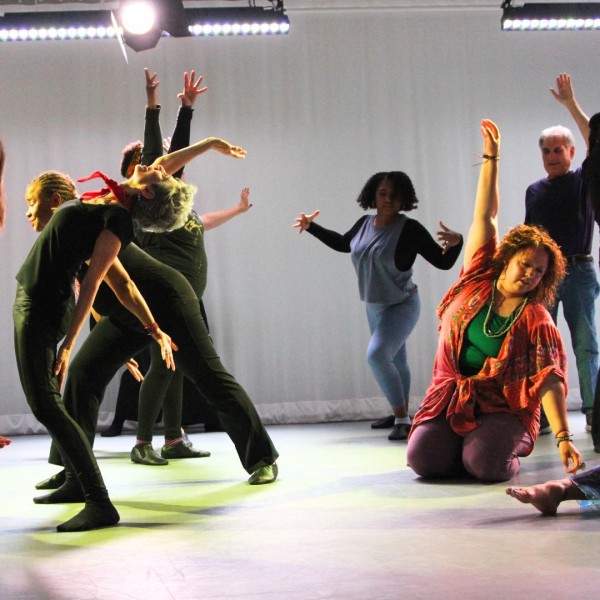In the photograph, a diverse dance troupe is captured mid-performance on a brightly lit stage that could very well be a dance studio. The setting is illuminated with a combination of powerful strobe lights and colorful lighting, casting yellow and pink hues on the polished white floor and projecting green shadows, subtly suggesting the presence of green disco lights. Behind the performers, a white curtain serves as a backdrop, and above them, track and theater lights shine down, adding to the vibrant atmosphere.

The dance troupe comprises approximately ten individuals of various ages, races, and genders, all adorned in multicolored costumes. Some performers wear dance shoes, while others are either barefoot or in black socks, emphasizing the casual and eclectic nature of the group. The troupe’s attire stands out, with one notable performer—a woman with long brown hair—wearing a red button-up blouse over a green shirt, paired with purple pants and a beaded necklace. She is positioned on the floor, her right hand lifted gracefully while her left hand reaches towards the ground. 

Around her, other dancers are caught in dynamic poses: a woman in the front arches her back, gazing upward, while another kneels forward behind her. A man stands behind the central woman with his hands raised, and another male dancer in the background extends his arms toward the sky. An African-American woman, with her hair in braids, wears a gray tank top over a long-sleeved black shirt and looks poised to perform a dance maneuver, appearing ready to move between the groups on either side of her. The scene captures a moment of diverse individual expression unified within a single vibrant performance.